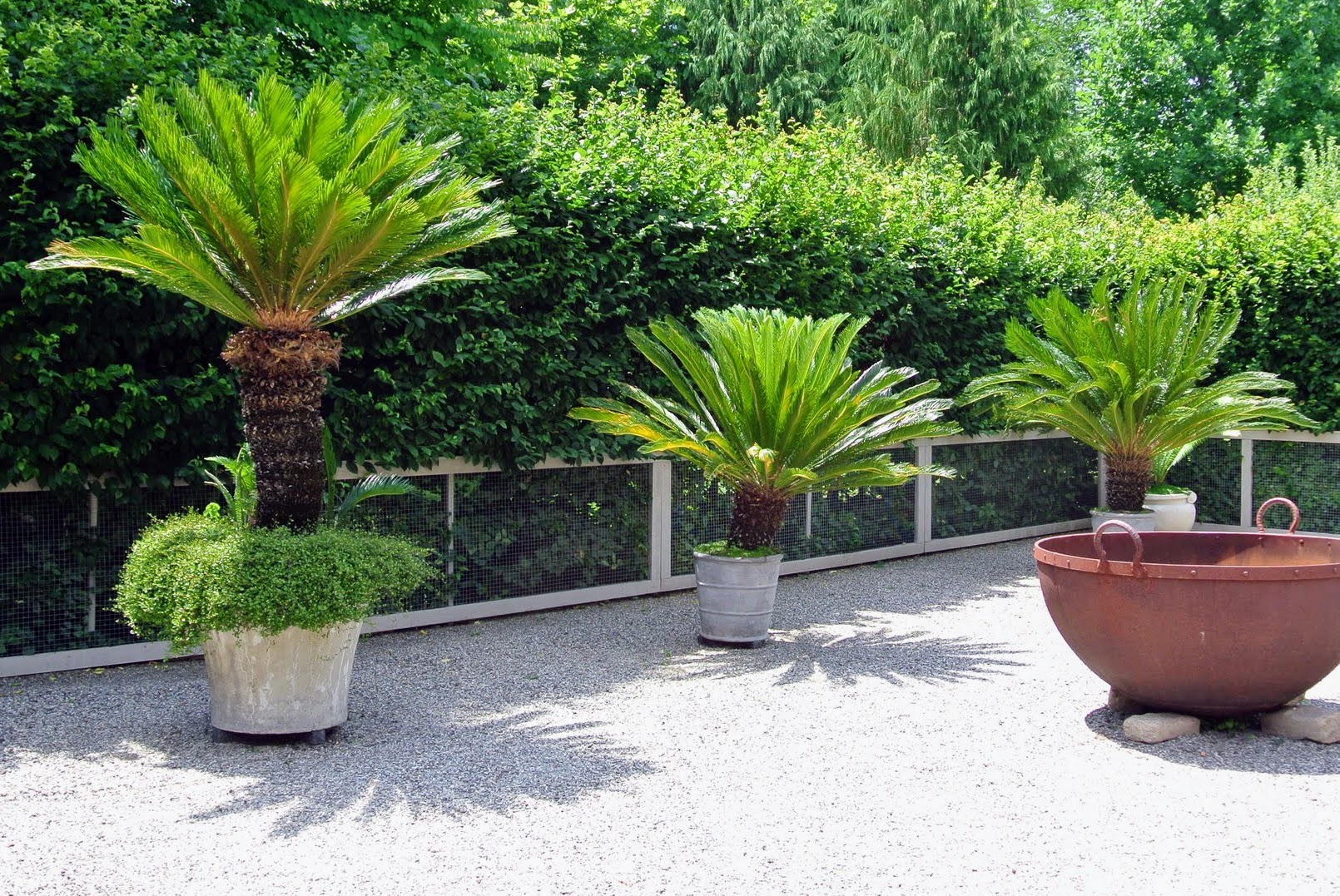The image depicts an outdoor garden or patio area with fine, light gray gravel covering the ground, extending diagonally from the bottom left to about a third of the way up the right side. Bordering the area is a short, white frame fence with netting and rectangular panels. Inside the fenced area, there are three young palm trees of varying heights planted in different containers: one in a large, gray concrete planter on the left, the second in a smaller concrete pot in the middle, and the third in another slightly larger concrete container on the right. Behind these, there is a white pot with a long, leafy plant. Additionally, a round, reddish metal bowl with two handles, possibly a fire pit, sits in the middle area, supported by white stone blocks. The background showcases a serene setting of tall green trees and various bushes, enhancing the garden feel of the space.